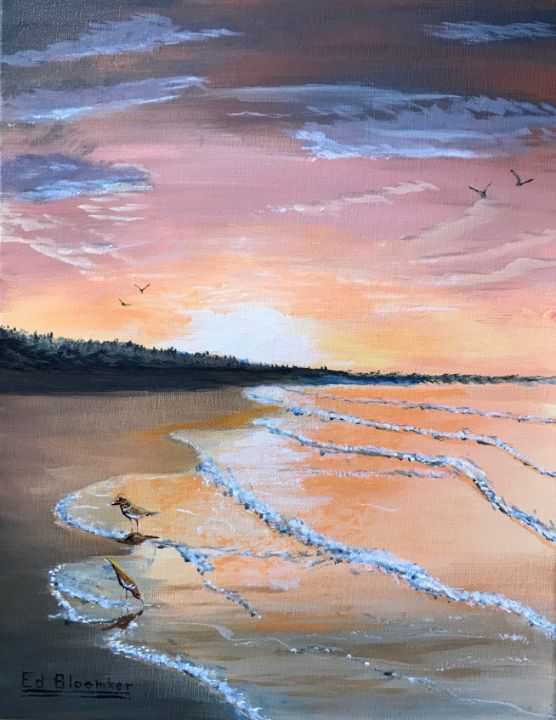This oil painting, possibly by artist Blomker as suggested by the signature "Blomker" in the bottom left, features an abstract but vividly colored beach scene at sunset. The beach, with its brown sand, stretches from the foreground towards the distant grassy hills in the background. The calm, foamy waves lap gently against the shore, dominating nearly half of the painting. In the background, dark gray grasses stand tall, silhouetted against the vibrant sky.

The sky itself is a stunning blend of rich peachy pink, yellow, and orange hues radiating from a bright white sun that sits close to the horizon. Further up, the sky hosts dark gray clouds, adding depth to the scene. Birds bring life to the composition—several sandpipers stand at the water's edge, while four seagulls soar above. The overall scene is serene and captivating, capturing the tranquil yet colorful essence of sunset at the beach.